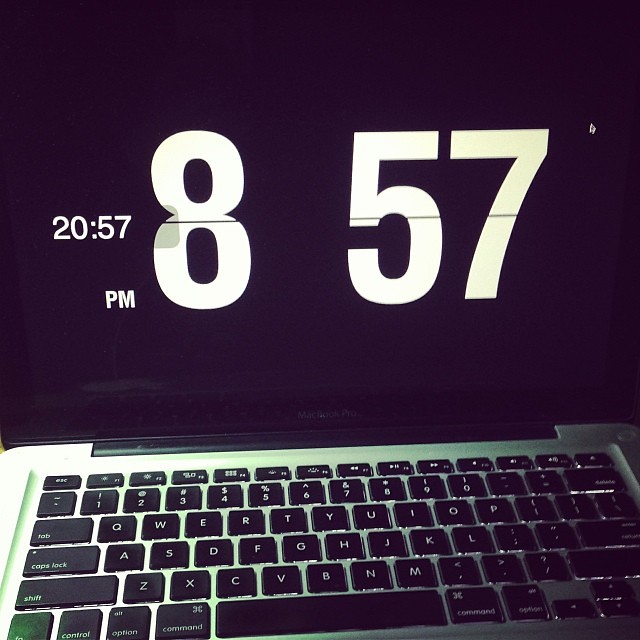The image depicts a green-colored laptop whose screen displays a black background with the time prominently shown. The time reads 8:57 p.m., with an additional military time format of 20:57 in smaller letters next to it. The digits of the time are segmented horizontally, resembling the flipping mechanism of a vintage Rolodex card. Beneath the time, although faint, the words "MacBook Air" can be discerned, suggesting the make and model of the laptop. The overall appearance of the laptop and the clarity of the screen imply it is a high-resolution, lifelike photograph.